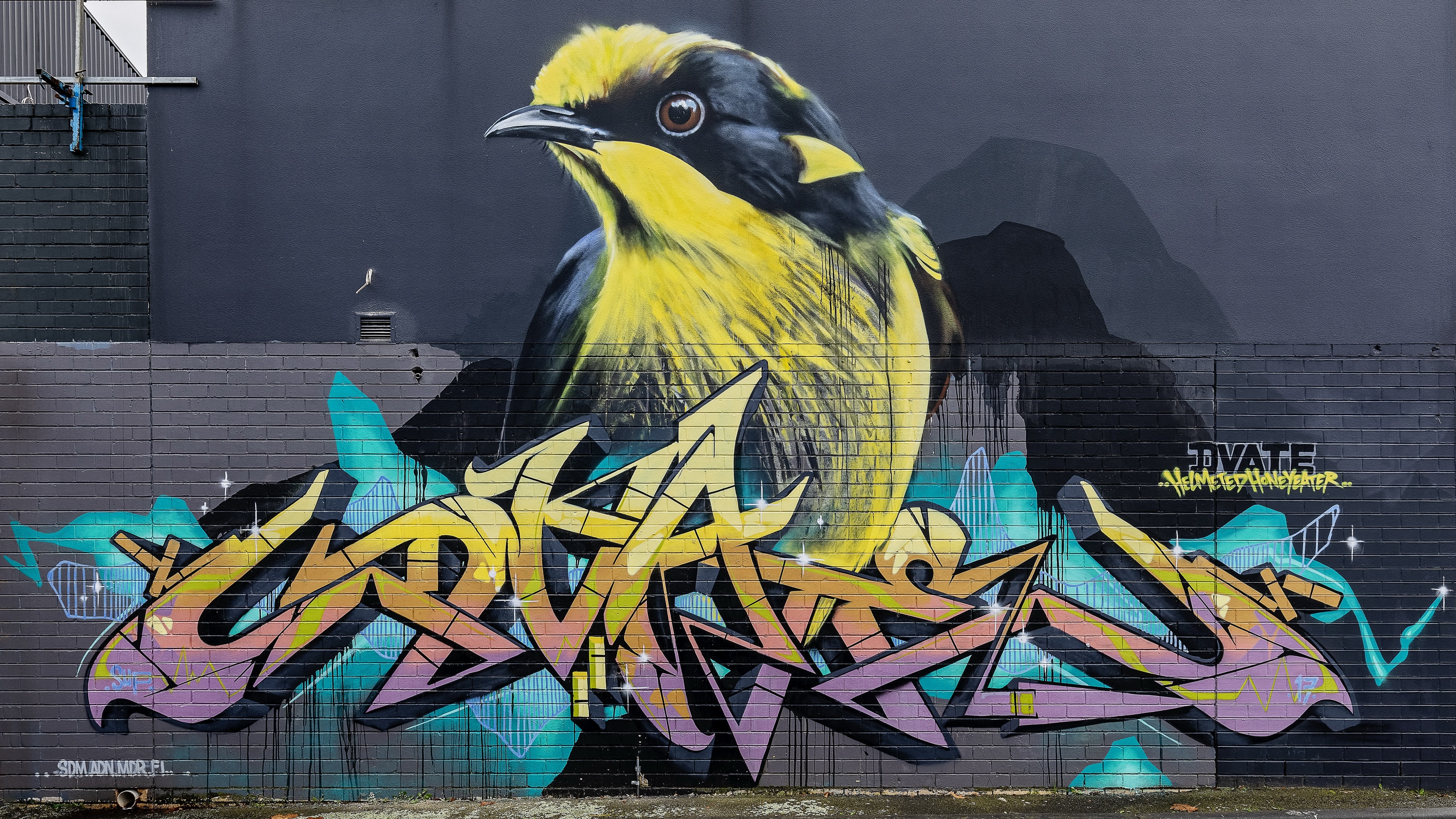The detailed graffiti painting on the side of a building features a vibrant bird with a yellow breast and a yellow stripe on top of its head. The bird, with its striking black wings, tail feathers, and body, points left, showcasing a shiny black beak and a distinct black swath around its eye. The background of the artwork consists of a brick wall, where the bottom part is a tannish color transitioning into a deep blue towards the top. Just above and to the left of the bird, there is a barred window, enhancing the urban feel of the scene. The wall behind the bird appears to be purplish and dark bluish, adding to the dynamic appearance of the artwork. There are vibrant, angled letters in purple, pink, yellow, orange, and light blue beneath the bird, indicative of the artist's tag, although they’re unreadable. Additionally, a smaller indication on the right-hand side reads "Teviot," with another signature in yellow below it.